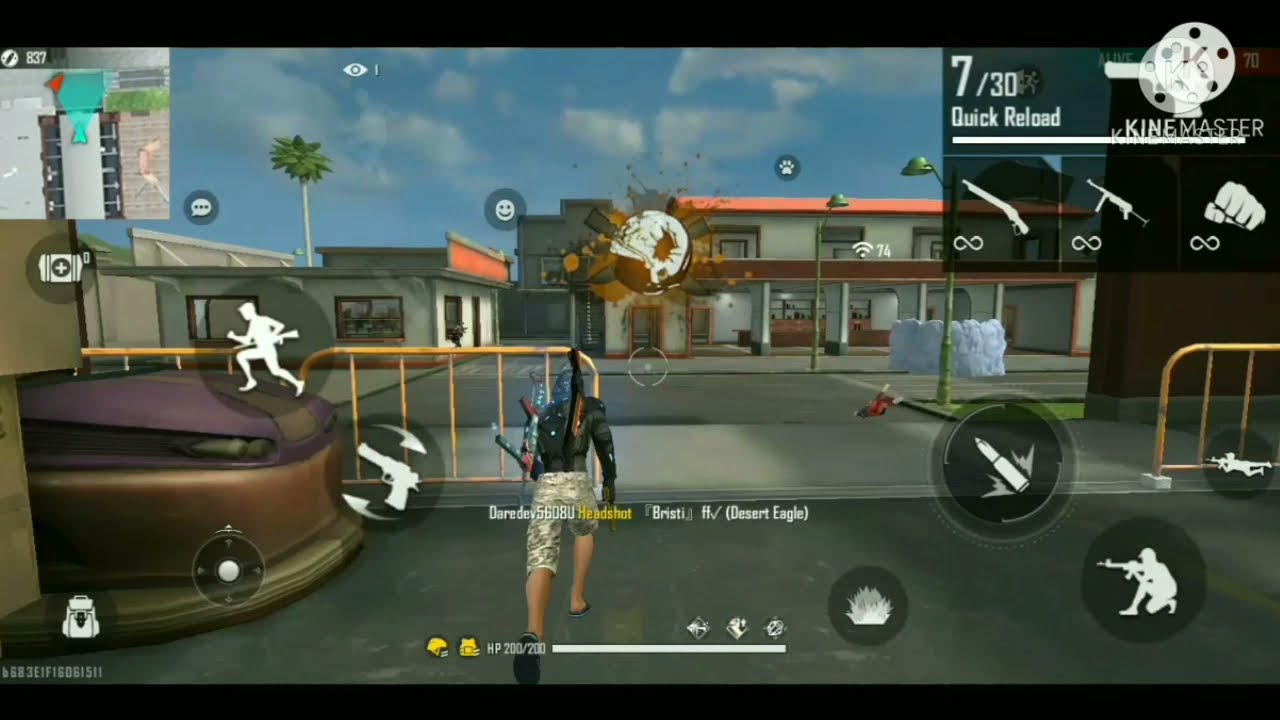This image is a detailed screenshot from a third-person action video game, likely showcasing a segment of intense gameplay. The central character, who appears to be the game player, is running forward, equipped with a quiver and an assortment of weapons, including a firearm. The character is distinctively dressed in camouflage knee-length shorts or possibly zebra print shorts, a black jacket, and what seem to be loafers or slippers.

The scene unfolds in what looks like a village plaza or a concrete yard, surrounded by buildings that resemble a hacienda, motel, apartment complex, factory, or warehouse. The environment has elements indicating recent or ongoing combat, such as explosions and barricades. There are multiple in-game icons scattered across the screen, including identifiers for a rifle, handgun, ammunition, medkit, and various action buttons such as crouch, quick reload, switch weapon, and others. 

In the upper right corner, the text reads "7/30 Quick Reload," accompanied by the KineMaster logo—a wheel of film, indicating this might be a recorded gameplay or edited video. Additional details include icons for crouching and shooting, indicative of the game's tactical depth.

In the background, silhouettes of armed men in motion further emphasize the game's action-driven narrative, while specific icons like a mini-map and a spread button highlight the game's interactive and strategic elements.